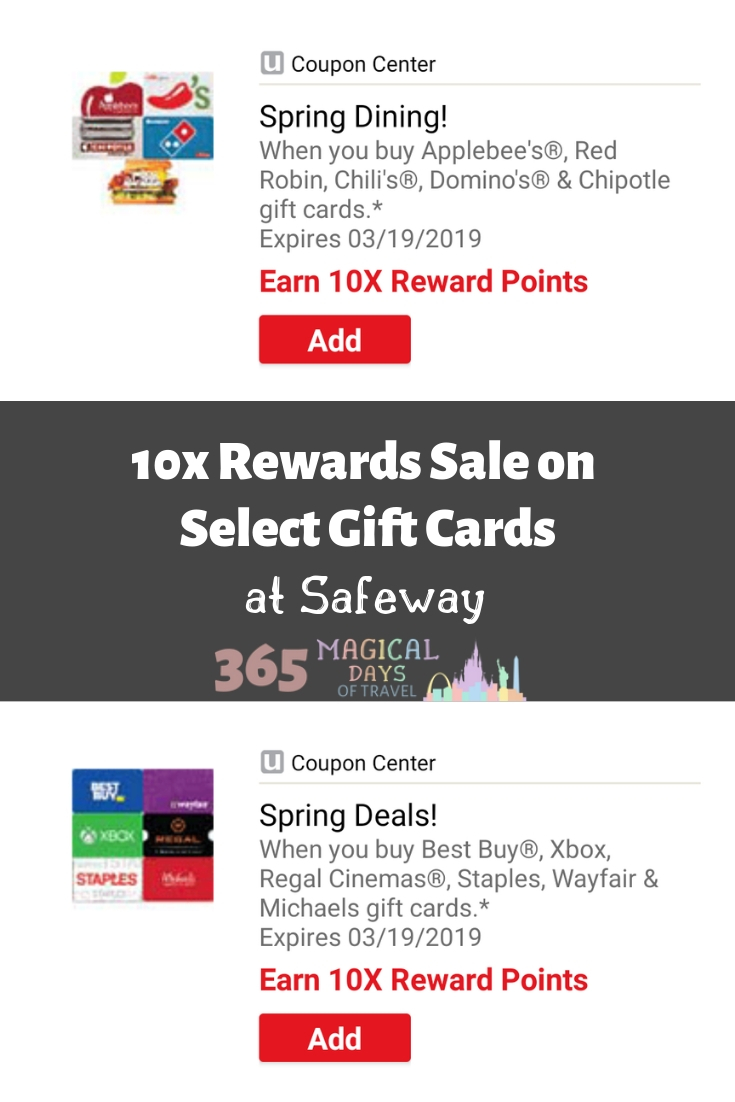The webpage displays a variety of gift cards and promotional messages, segmented into different sections. 

On the left-hand side, there are images of gift cards for Chili's, Applebee's, an unidentifiable card, and Domino's, along with what appears to be a sub sandwich.

On the right-hand side, there is a gray square with a white "U" logo labeled "Coupon Center." Below this, the headline "Spring Dining!" in bold black text is followed by detailed information in regular black or dark gray text: "When you buy Applebee's, Red Robin, Chili's, Domino’s, Chipotle gift cards *Expires 03-19-2019.” Highlighted in red, it states, "Earn 10x Rewards Points," referring to earning ten times the usual rewards points. There is a clickable red rectangular button with white "Add" text.

Further down, there is a prominent dark gray rectangular area with bold white text: "10x Rewards Sale on select gift cards 10x at Safeway." The word "Safeway" is italicized. Below this, in multicolored text, the message "Magical Days" is spelled out: "M" in purple, "A" in red, "G" in orange, "I" in yellow, "C" in green, "A" in blue, "L" in purple, "D" in red, "A" in orange, "Y" in yellow, "S" in green. There is an illustration of a multicolored castle in purple, green, yellow, blue, orange, and pink.

Another section displays further gift cards including Best Buy (in purple), Xbox, Regal Cinemas, Staples, and possibly Hallmark. The section is labeled "Coupon Center, Spring Deals!" followed by information in bold gray text: "When you buy Best Buy, Xbox, Regal Cinemas, Staples, Wayfair, Michaels gift cards *Expires 2023/19/2019.” In red text, it says "Earn 10x reward points." There’s another red rectangular button with white text that says "Add."